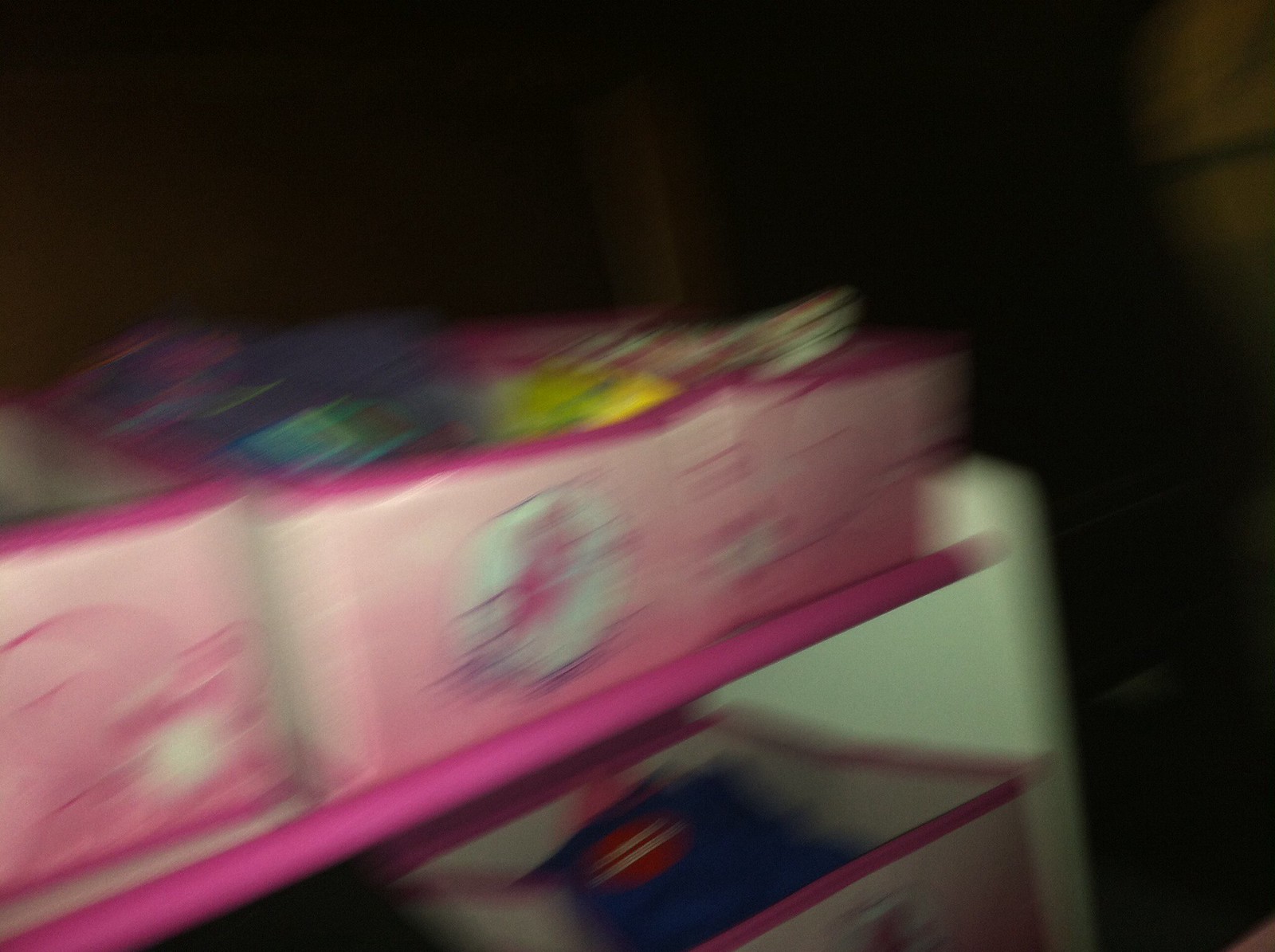The image is a blurry photograph, likely taken with the camera in motion, depicting a distinct shelving unit. The shelves, which appear to be purplish or pink, have white edges. At least three pink rectangular fabric boxes, possibly with a character or logo on the front, are placed on the shelves. The top box, containing what seems to be clothes or toys in shades of yellow, purple, and white, sits prominently. Directly below it, another box holds items that display a mix of blue, red, and yellow colors. The background is predominantly black, slightly revealing a wooden beam and a yellowish object to the right. Overall, the image conveys a sense of childlike or playful storage, potentially in a toy display, hampered by blurriness and motion blur.